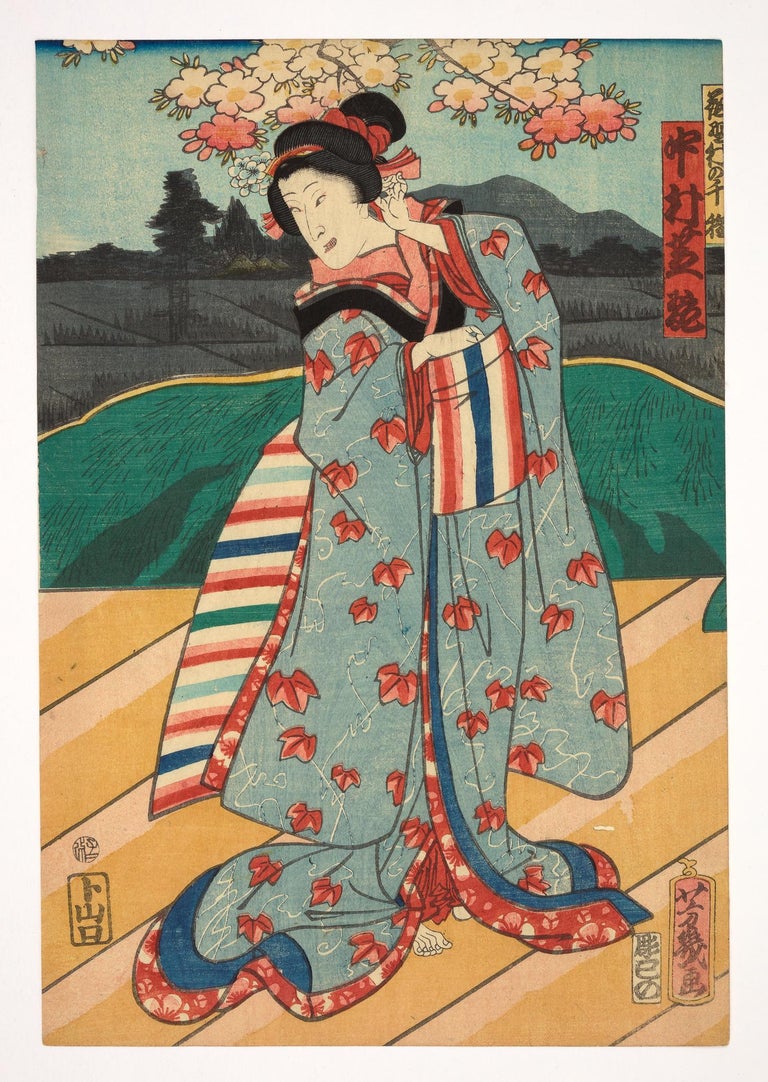This detailed Japanese illustration depicts a woman, possibly a geisha or a Kabuki character, dressed in a vibrant kimono. The kimono is primarily blue, adorned with wavy white lines and red maple leaves, and cinched with a striped belt. Her hair is styled in a topknot, secured with a red sash and a comb above her forehead. The woman holds her hands near her waist and head, while she gazes downward at the ground or her dress.

She stands on a surface with diagonal beige and orange stripes, possibly a wooden flooring next to a body of water. In the background, a serene landscape features elements such as cherry blossoms at the top, green grass, and a distant mountain surrounded by trees and fields tinged with dark red hues. Two Japanese calligraphy banners are positioned on the right: a larger red one lower and a smaller yellow one near the edge of the frame. A yellow band runs horizontally from left to right, forming a shape that resembles a low hill or mound.